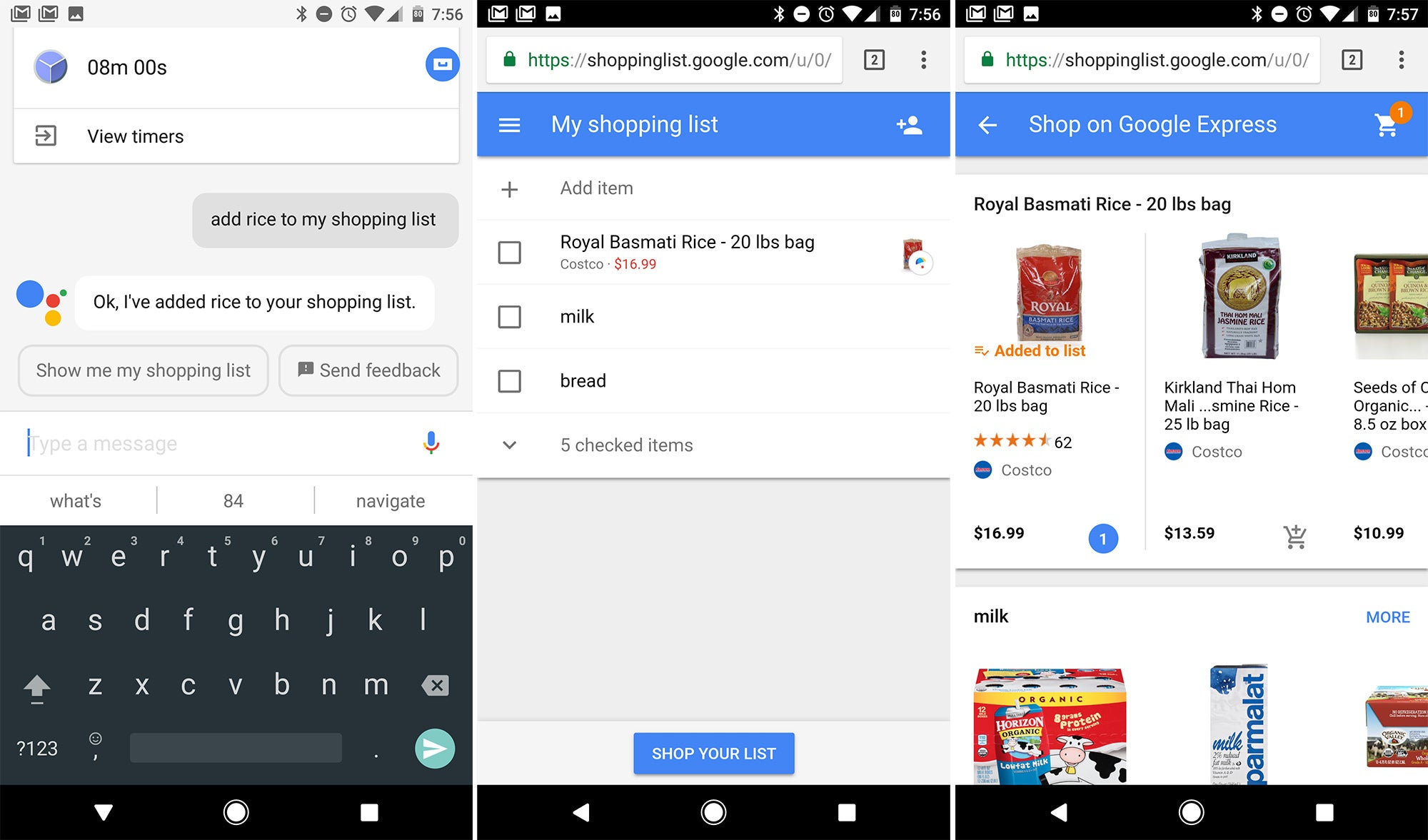The image consists of three sequential screenshots from a smartphone screen, illustrating a voice-command interaction and subsequent actions. 

In the first screenshot, the time displayed in the upper right-hand corner is 7:56. A small blue circle with the text "8 minutes 0 seconds" is visible, likely indicating the current duration of an ongoing activity. The primary content of this screenshot includes a speech bubble that reads, "Add rice to my shopping list," with a subsequent response bubble stating, "OK, I've added rice to your shopping list." The on-screen keyboard is also visible at the bottom, suggesting active input.

The second screenshot displays the content of the shopping list. The URL "https://shoppinglist.google.com/.u/.o/" is shown in the address bar. A blue bar at the top of this screenshot reads "My Shopping List," clearly identifying the list's purpose. Below the blue bar, several items are displayed with corresponding checkboxes for each, allowing for item management on the list.

In the final screenshot, the time has progressed to 7:57. The top blue bar now states "Shop on Google Express," accompanied by a shopping cart icon and an orange circle with the number 1, indicating a notification or item count. The screen displays three images of different types of rice at the top and below them, three images of various milk products, showcasing shopping options relevant to the user's previous voice command.